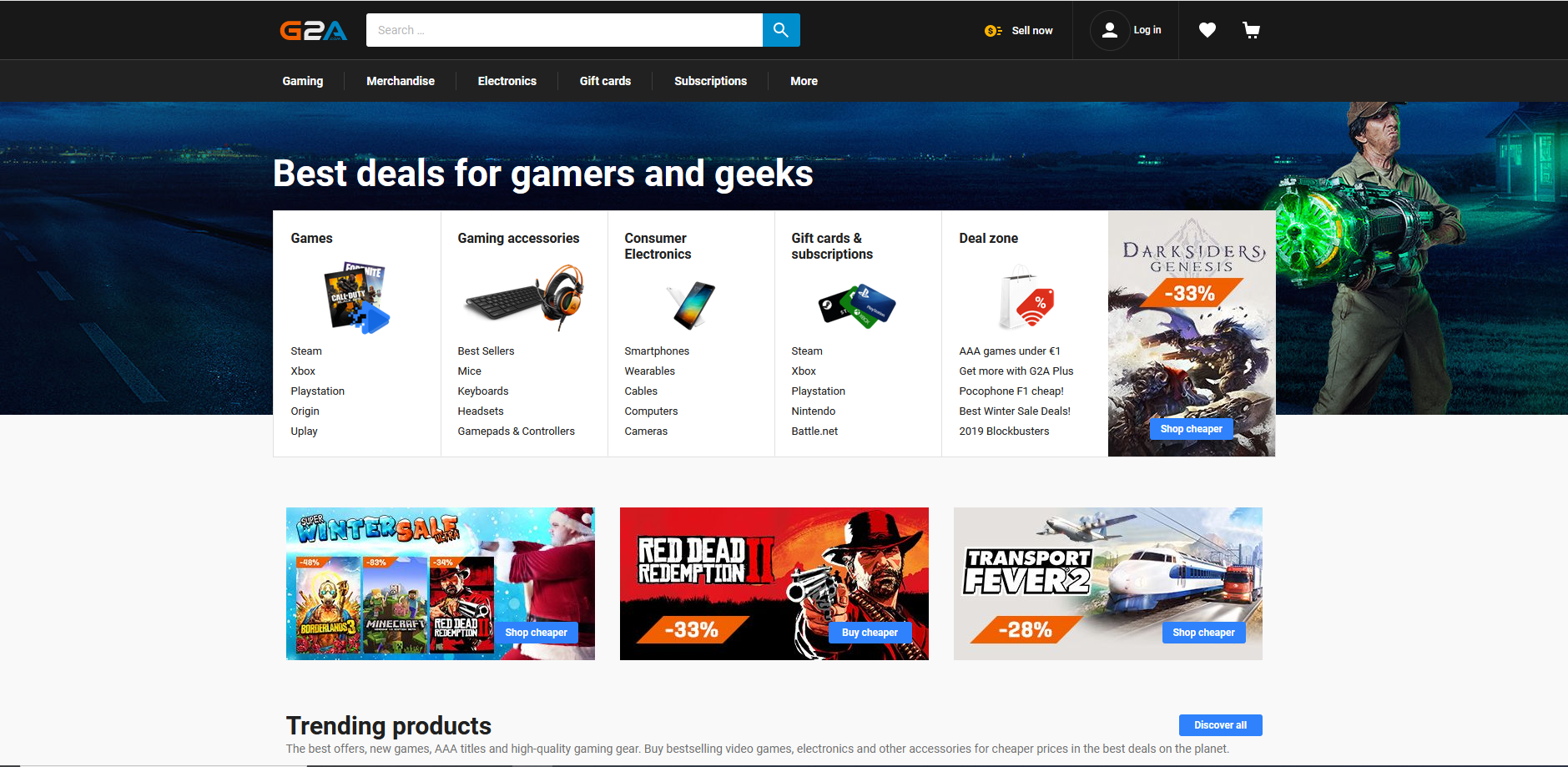This is a detailed screenshot of a gaming website named G2A. The site's logo, located at the top-left corner, features a stylized 'G' in orange, '2' in white, and 'A' in blue. A black navigation bar spans the top of the page, immediately right of the logo, there's a search bar for quick access. At the top-right corner, options for user interaction are visible: a "Sell Now" button accompanied by a golden money symbol, indicating a marketplace feature, a "Log In" button, a heart icon symbolizing a wishlist, and a cart icon for shopping.

Just below the top navigation, another menu offers categories like Gaming, Merchandise, Electronics, Gift Cards, Subscriptions, and a dropdown for more options. Beneath this menu, a prominent banner declares "Best deals for gamers and geeks," segmenting into different tabs: Games, Gaming Accessories, Consumer Electronics, Gift Cards & Subscriptions, and Deal Zone.

On the right side of the main banner, an advertisement highlights "Darksiders Genesis," showcasing a 33% discount, with a blue "Shop Cheaper" button below. Further down, three more promotional ads are displayed: the "Winter Sale" in the bottom left, "Red Dead Redemption 2" at 33% off in the bottom middle, and "Transport Fever 2" offering a 20% discount at the bottom right. This screenshot effectively captures the essence of G2A's user interface and promotional offerings.